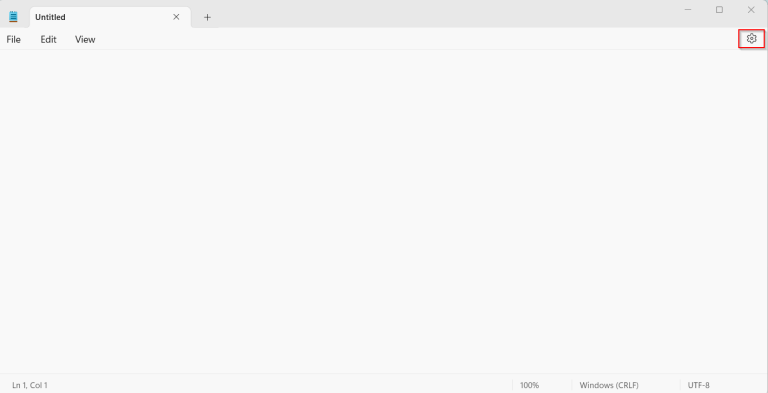This horizontal rectangular image primarily showcases an interface of a software window. The topmost section spanning from left to right is an off-white to light gray color. In the top left corner, there is a turquoise element connected to a bright white tab that displays the word "Untitled" in bold black font. To the right of "Untitled" there's an 'X' icon, and further to the right outside the tab is a plus sign.

Returning to the off-white/gray area on the right side, there are three icons arranged sequentially: a dash, a square, and another 'X'. Below this off-white/gray area, the rest of the screen is a crisp, bright white. On the left of this white area, in bold black font, are the words "File," "Edit," and "View," separated by spaces. A thin line runs horizontally under these words, stretching to the right edge of the image. On this same horizontal plane, at the right edge, is a gray settings button, outlined by a red horizontal rectangle.

At the very bottom of the screen, there is a thin horizontal line. In the lower left corner, the text "Ln1, Col1" is displayed in black font. Moving towards the center from the bottom edge, there is a "100%" indication. Further right, in gray font, the word "Windows" is written with "(CRLF)" in parentheses next to it. The text on the far right side of the bottom edge is not legible.